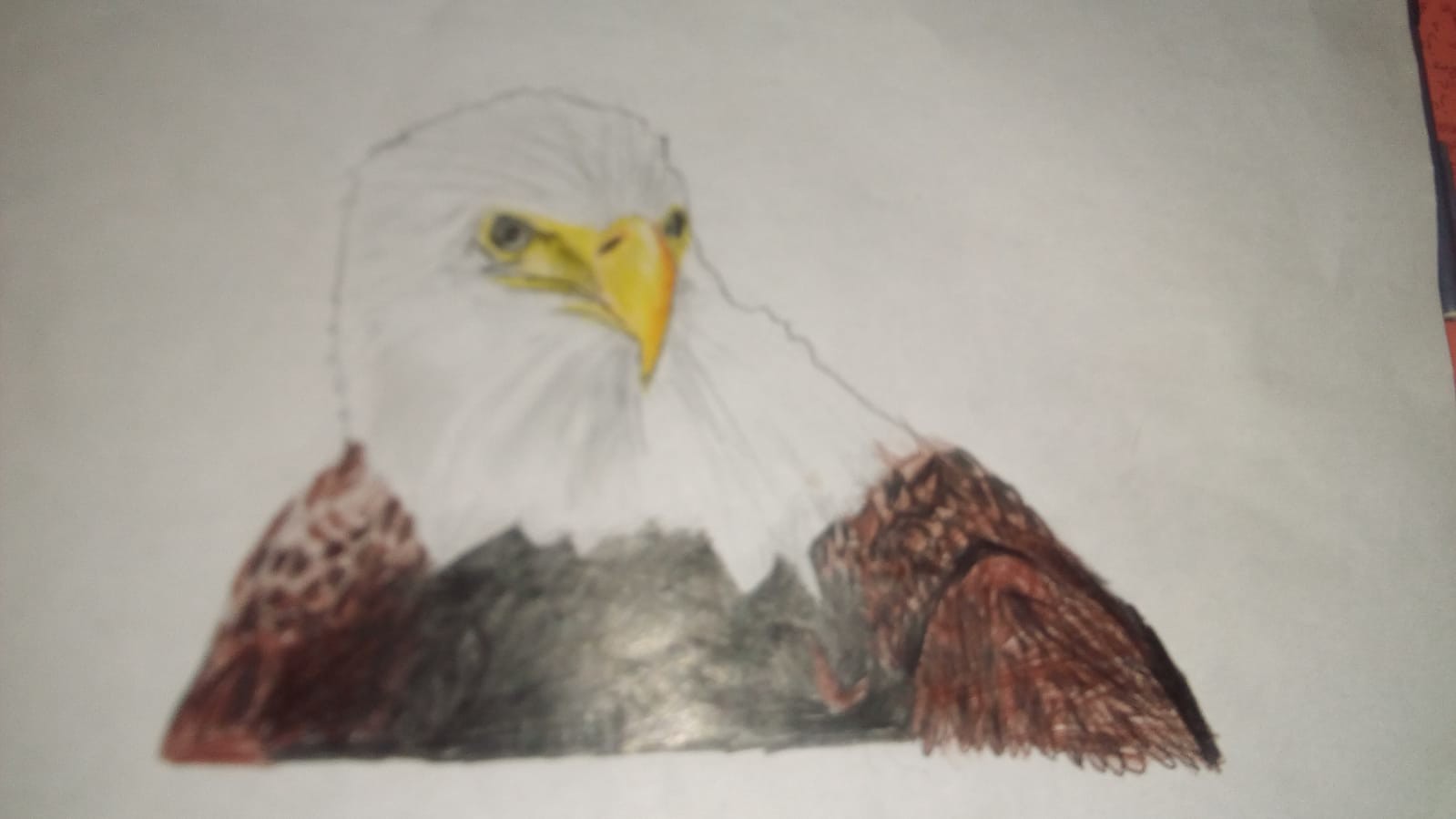This photograph showcases a detailed drawing on a pristine white piece of paper, laying on a polished mahogany or oak desk. In the top right corner of the image, a patch of color and a black area are visible, possibly part of the paper's border or an unrelated item on the desk. The central focus is a meticulously drawn bald eagle, characterized by its distinct white head and striking yellow beak. The bird's shoulders and upper wings display rich brown tones, although the term "fur" is more accurately feather plumage. The drawing extends slightly below the eagle's head and shoulders, revealing some black shading underneath but ending abruptly without showing the bird's full body or additional feathers. Rendered primarily in pencil, the drawing also incorporates strategic use of color, lending a lifelike quality to the eagle's features, including its piercing eyes. The overall composition is simple yet compelling, with the dark hues and fine details adding depth and realism to the artwork.